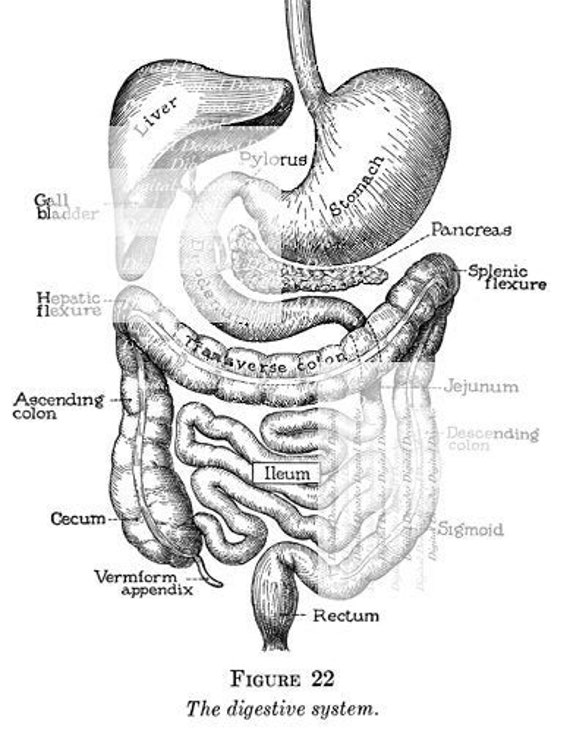This black and white scan appears to be an old-style anatomical drawing of the human digestive system, likely from an anatomy manual, displayed against a solid white background. The image prominently features the digestive organs with intricate sketches providing depth to each structure. Notable components include the liver at the top, followed by the pylorus, stomach, pancreas, gallbladder, and hepatic structures. The digestive tract is detailed from the esophagus down to the rectum, including the stomach, ileum (seemingly mislabeled as "heum"), ascending and descending colon, transverse colon, and splenic flexure. Semi-transparent white boxes with text partially obscure some details. The diagram is labeled "figure 22, the digestive system" at the bottom.